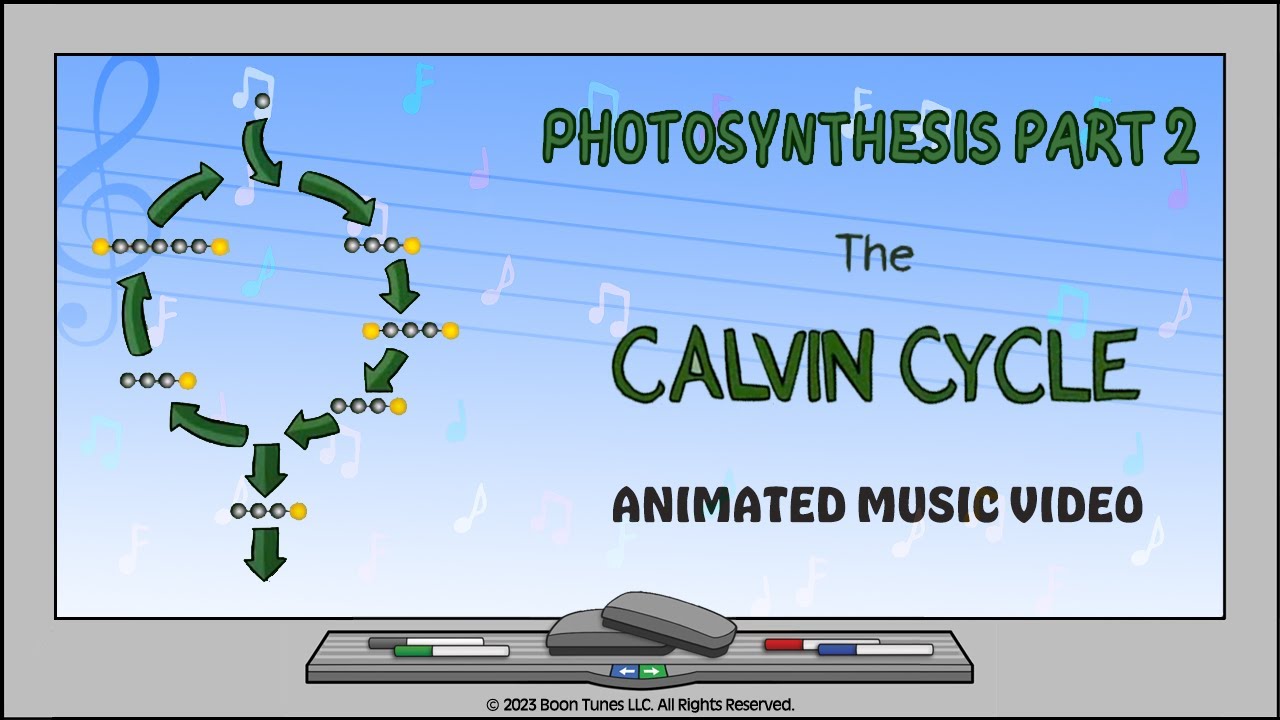The image is a detailed and animated scientific diagram of photosynthesis focusing on "Part 2, The Calvin Cycle." The central feature is a cycle comprised of green arrows arranged in a circular formation, illustrating each stage of the Calvin Cycle. Along these arrows are several grey dots, one of which is gold, representing different steps in the photosynthesis process. The drawing is set against a dry erase board, characterized by its blue and white background filled with scattered musical notes in blue, pink, and white, suggesting a musical element tied to the animation. 

The dry erase board has a defined outline with a gray middle bordered by two thin black lines. At the bottom, there are four marker pens: a gray-capped marker, a green-capped marker on the left, and a red-capped marker, along with a blue-capped marker on the right. Also present are a blue arrow pointing left and a green arrow pointing right, likely indicating navigation controls. The text on the image includes "Photosynthesis, Part 2" written in green in the top right corner, followed by "The Calvin Cycle" in green, and "Animated Music Video" in black beneath it. At the very bottom, the caption "Copyright 2023, Boone Tunes, LLC. All rights reserved." indicates ownership and rights to the content. The overall presentation suggests that this image might be a static capture of an animated music video that educates viewers on the Calvin Cycle of photosynthesis.